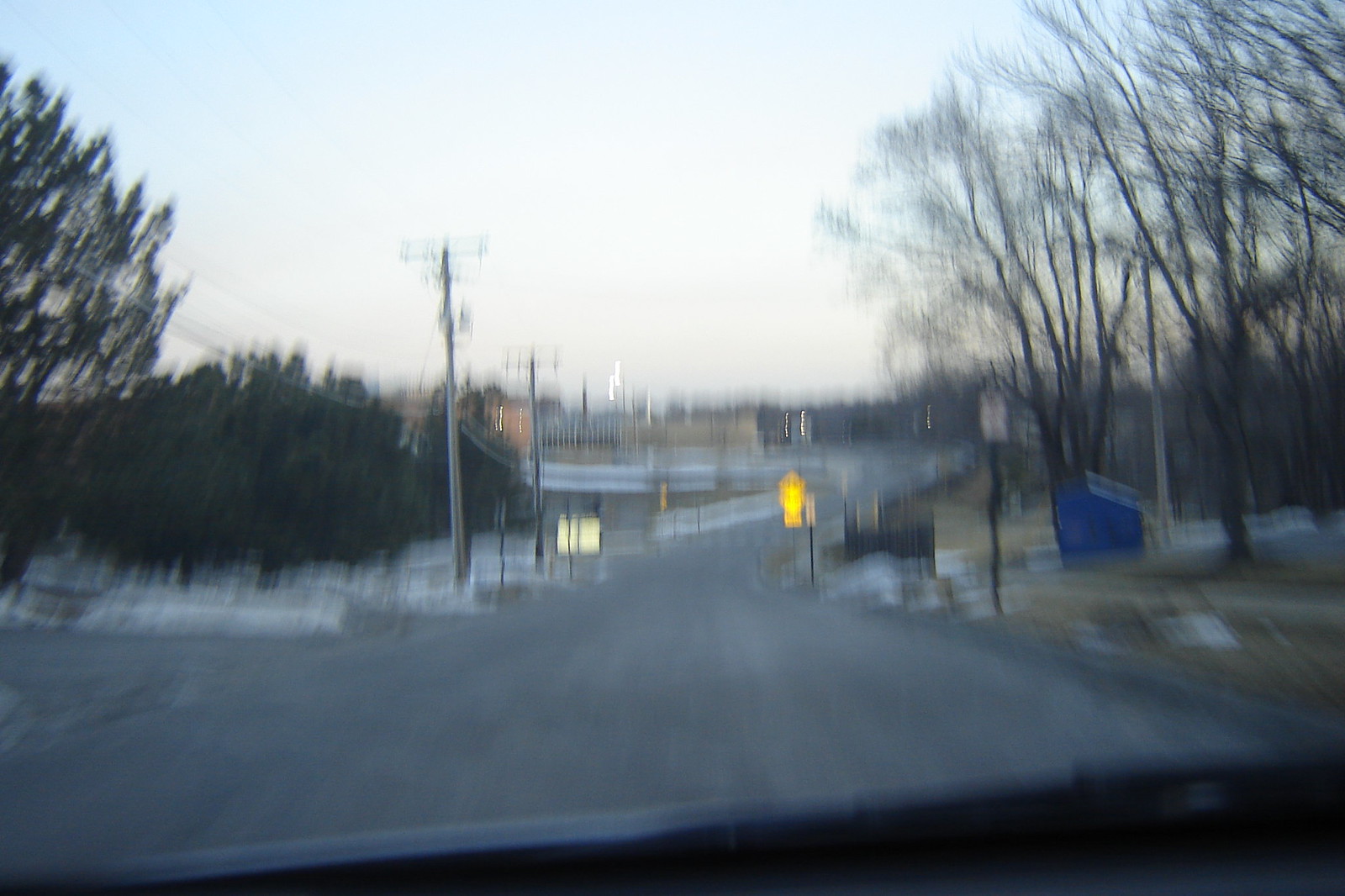The image depicts a downhill, wide road with no visible road markers. There's a prominent "No Parking" sign, likely in red and white. A blue object, possibly a dumpster or small shelter, is also present. White fences line the road, which is flanked by trees on both sides. Telephone poles march down the road's length. In the distance, the road curves sharply to the right, with white fencing marking the turn. Beyond the turn, there seems to be a school or similar structure. The scene is set under a gray, cloudy sky.